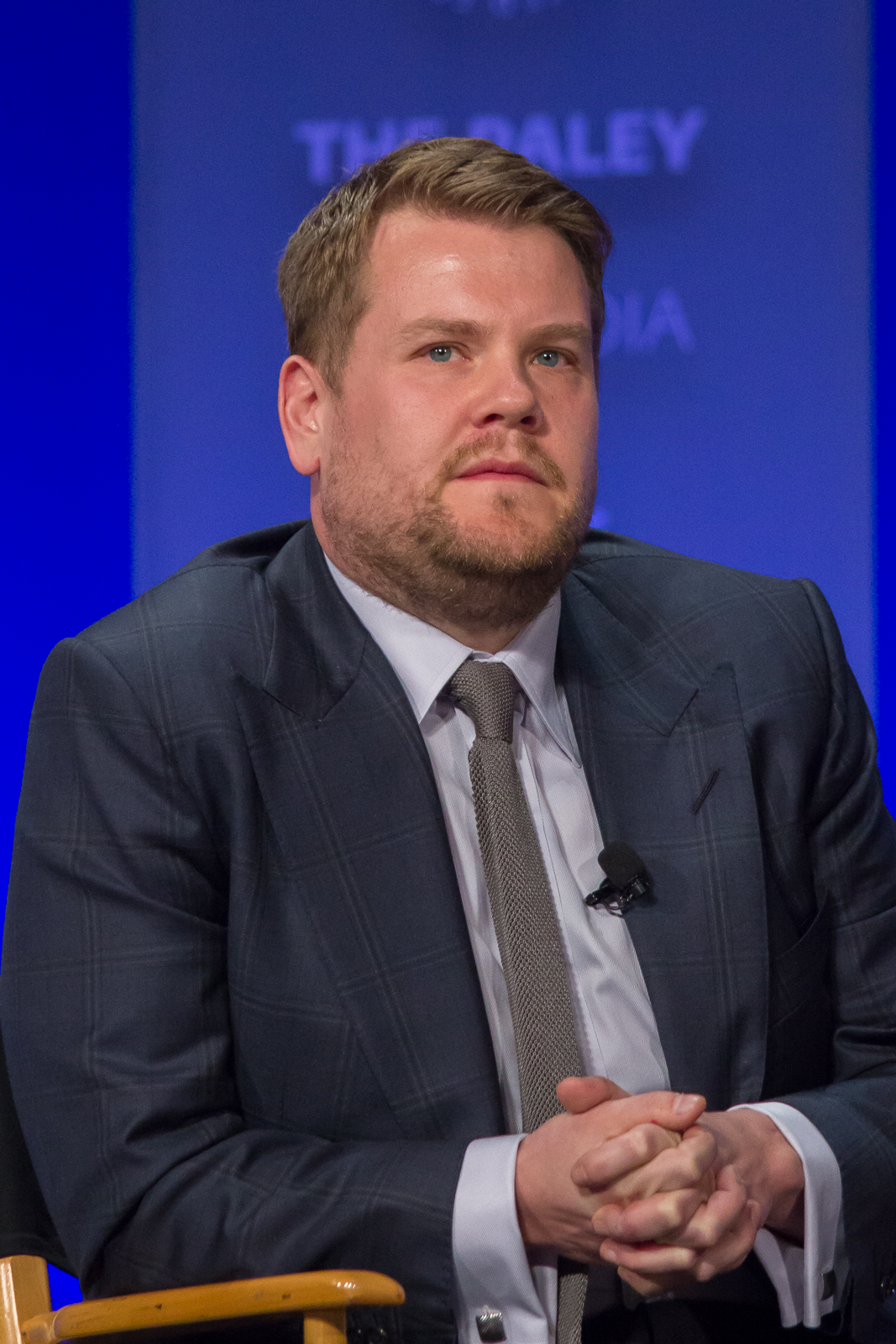The photograph features a white male with reddish-brown, light brown hair, and stubble matching his hair color. He has striking baby blue eyes and a composed expression. He is dressed in a sophisticated dark blue business suit, complemented by a light gray button-down long-sleeved collared shirt with cufflinks on the sleeves, and a dark gray tie. A microphone is clipped to the blazer, indicating a formal setting or interview. His hands are folded together in his lap, fingers clasped.

He is seated in what appears to be a brown and black director's chair, with a visible wooden armrest on the left side of the image. The backdrop features a bright blue wall with partially legible large capital letters above his head, spelling "THE DAILY" (or a similar phrase). The composition and details suggest a professional or media-related environment.